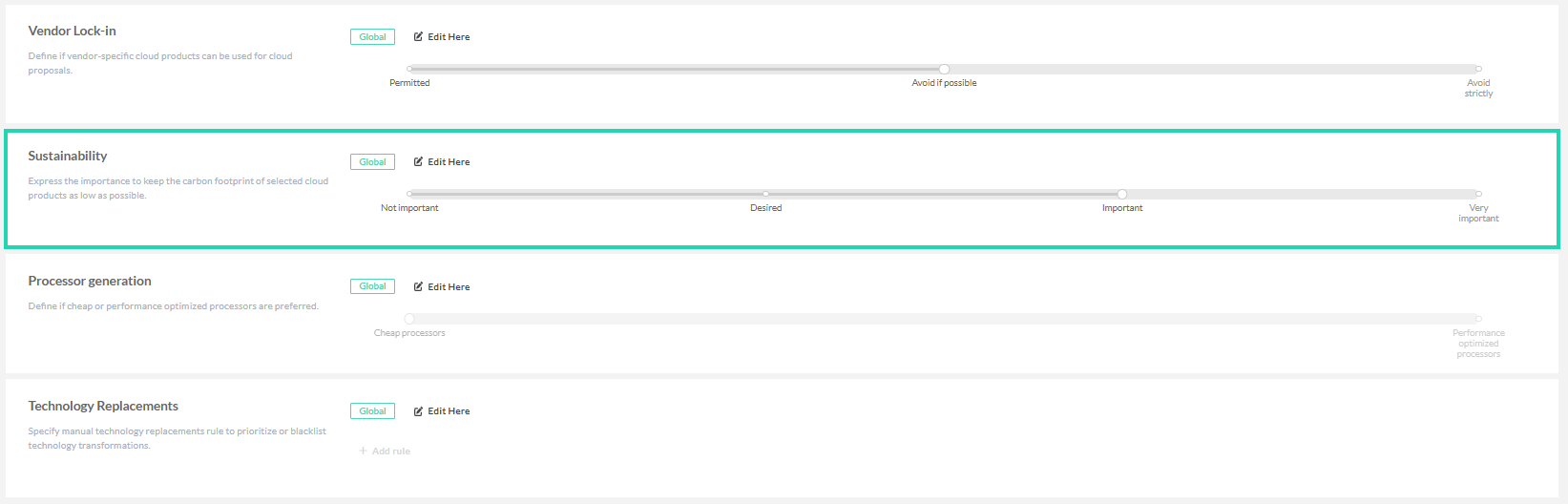This horizontal image features a pale light gray border and is divided into four equal sections by thin gray lines. Each section is labeled on the left side with the following headings: "Vendor Lock-In," "Sustainability," "Processor Generation," and "Technology Replacements." Beneath each heading, there is a small area of light gray text.

On the right side of each section is a thin font button outlined in blue and green, labeled "Global." Next to this button is a "Edit Here" option accompanied by a checkbox.

The top two sections, "Vendor Lock-In" and "Sustainability," each contain a slider. For "Vendor Lock-In," the slider ranges from "Permitted" on the left to "Avoid If Possible" in the center, and "Avoid Strictly" on the right. The "Sustainability" section’s slider is outlined in aqua green and spans from "Not Important" on the left, to "Desired," "Important," and "Very Important" on the right.

The "Processor Generation" section also has a slider, although it is very light. The slider ranges from "Cheap Processors" on the left to "Performance-Optimized Processors" on the right.

The bottom section, labeled "Technology Replacements," does not feature a slider.